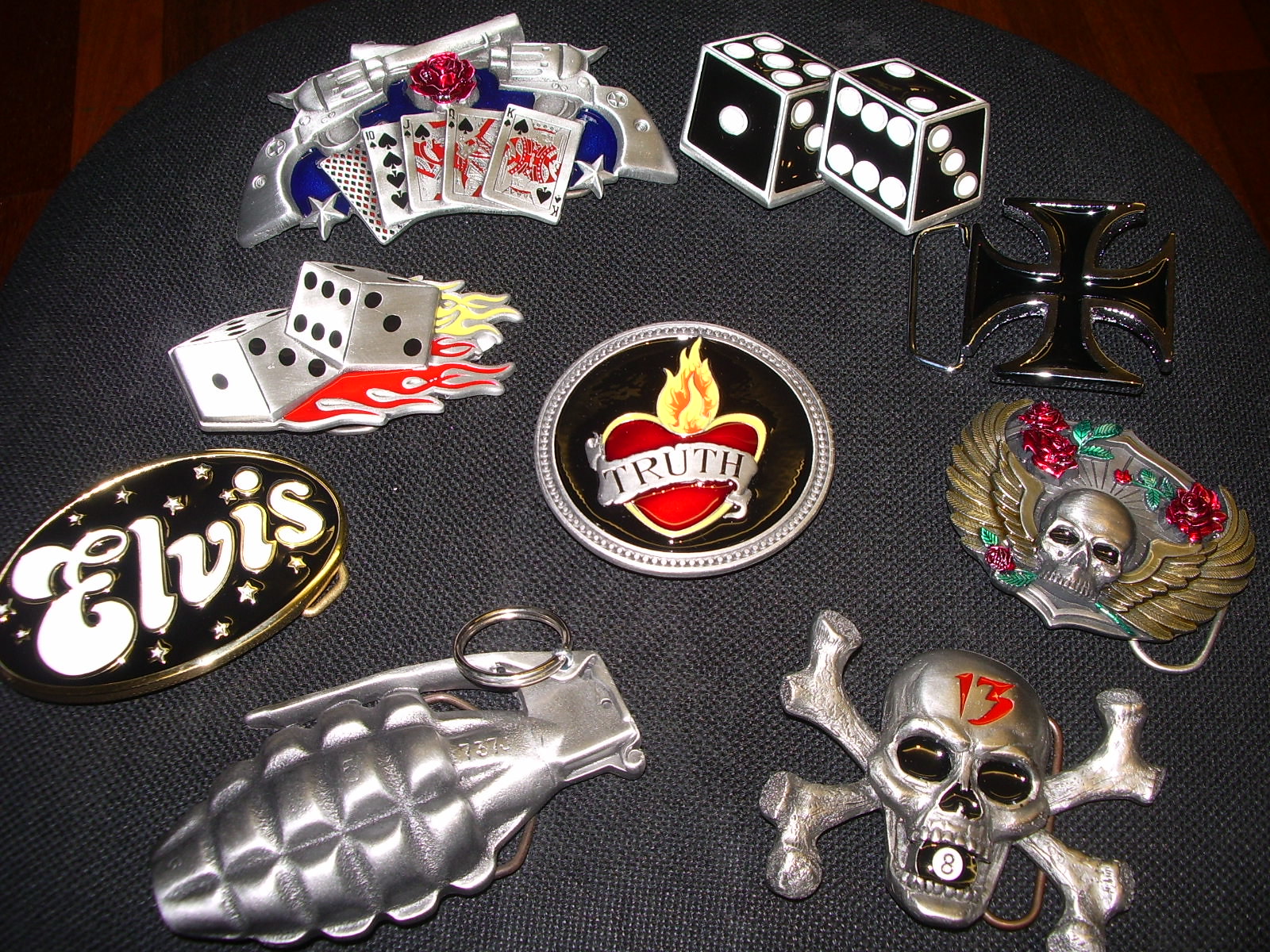In the photograph, set against rich, dark brown, and reddish hardwood floors, lies a black, rough canvas fabric adorned with a collection of intricately decorated belt buckles and keychains. Each item adds a vibrant story to the ensemble.

Starting from the bottom left, there is a small, realistic silver metal grenade that appears to be a keychain, complete with the number 737 and a silver key ring. Above it, a magnet or buckle showcases a black surface with gold trim, white stars, and the name "Elvis" boldly written in white text.

Moving upwards, there is a dynamic pair of white dice with yellow and orange flames shooting up from them, depicted mid-motion; one die shows a 1 and a 3, while the other displays a 6 and a 3. Adjacent to this is a captivating emblem featuring a poker hand consisting of a straight flush—10, Jack, Queen, King, and Ace of spades—framed by two silver stars and crowned by crossed silver revolvers with a red rose accentuating the design.

Next, there are black dice, showing a 5, 1, and 6 on one and a 6, 3, and 2 on the other, followed by a distinctive iron cross buckle, outlined in silver and black in the center.

In the middle of this collection, a standout silver circular emblem features a black background, with a striking red heart at its center. Flames rise from the heart, which is encircled by a banner displaying the word "Truth."

Towards the bottom, there is a formidable silver skull with a menacing 8-ball lodged in its open mouth and the number 13 inscribed in red on its forehead. Its eyes are dark and haunting. Another striking piece, nearby, shows a silver skull with golden wings, clenched between its teeth is a red rose with a green stem, flanked by red and green floral designs.

This detailed collection of emblems and buckles, each with unique themes ranging from iconography, gambling elements, and classic rock references, is vividly showcased on the rich wooden floor backdrop.